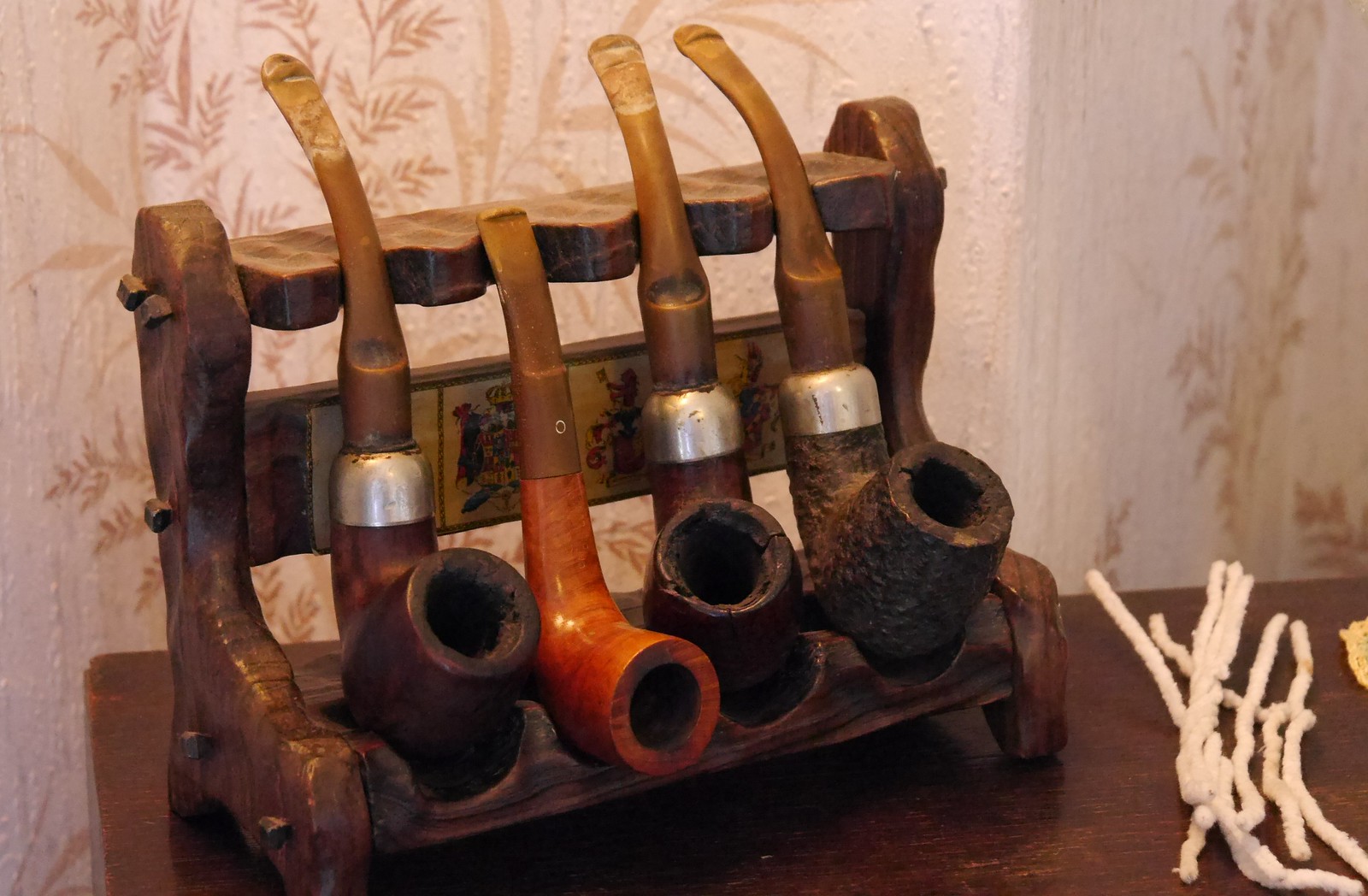In this detailed photograph, four smoking pipes are meticulously displayed on a hand-carved wooden stand, designed specifically for showcasing these pipes. The stand itself, which appears to be handmade, features intricate carvings and exudes a rustic charm. The pipes, each varying in shape, size, material, and color, are aligned from left to right. The first pipe is a long wooden one with a rich brown hue. Next, there's a lighter brown pipe, seemingly crafted from horn. The third pipe returns to a wooden design, slightly more reddish in color, and the final pipe is uniquely carved from stone, exhibiting a weathered appearance. This elegant display is set against a backdrop of wallpaper adorned with a subtle tree and leaf pattern, and the stand rests upon a wooden table. In the lower right corner of the image, some white pieces of string are visible, adding a touch of everyday realism to the scene.